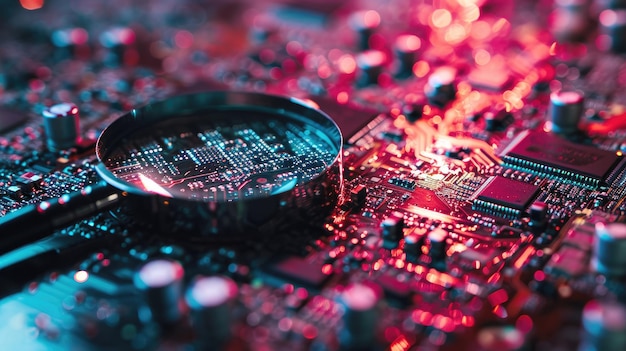This professionally taken, color photograph in landscape mode showcases a highly detailed, close-up view of a complex microchip or circuit board. Shot from just above, looking down at a diagonal angle, the focal point centers on the intricacies of the panel, while the foreground and background blur into soft focus. The circuit board is dotted with an array of components, including numerous small metallic points, silver controls, and raised knobs, some of which could be turned or adjusted.

A magnifying glass, approximately four inches in diameter, rests atop the panel, offering a glimpse of the fine circuitry beneath its clear surface. Adding to the technological atmosphere, a red backlight bathes at least half of the circuitry, casting a warm glow over the scene. Accents of blue and various other colors speckle the field of vision, enhancing the detailed textures and lending a sophisticated, almost otherworldly feel to the circuitry. The composition, suggestive of an advanced instrument panel, switchboard, or potentially spacecraft controls, captures the meticulous and intricate inner workings of modern technology.